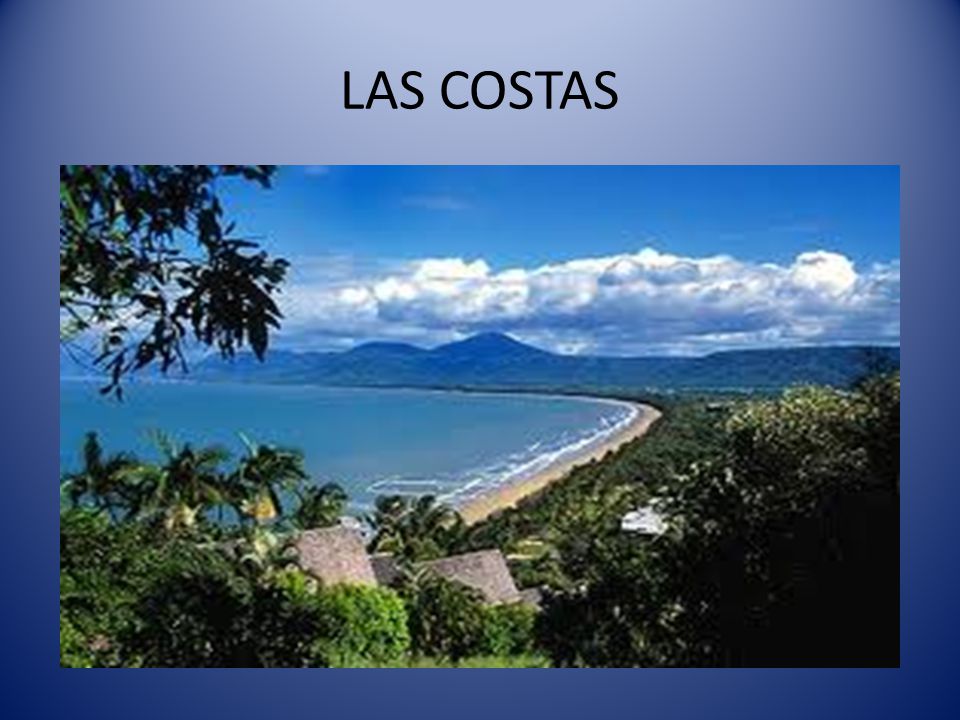The image features a postcard-style scene with a blue gradient background, transitioning from light blue at the top to dark blue at the bottom. At the top, the text "Las Costas" is clearly displayed in black, all-caps, sans serif font. The central photograph, slightly grainy and taken from an aerial perspective, overlooks a serene beach flanked by verdant forest on the right. The coastline curves in a U-shape from the bottom left to the middle, extending towards the upper left, where the sand meets the clear blue ocean. Waves ripple gently across the water, leading towards distant, green-covered mountains under a sky dotted with fluffy white clouds.

The immediate foreground reveals grey and beige rooftops of a couple of homes peeking through the dense palm trees and vibrant green foliage. Tree branches extend into the frame from the upper left, adding a layer of depth and enclosing the viewer within the lush tropical forest, looking down towards the tranquil coastline. Despite the idyllic setting, the absence of people on the beach lends a surreal quality to the picturesque vista.